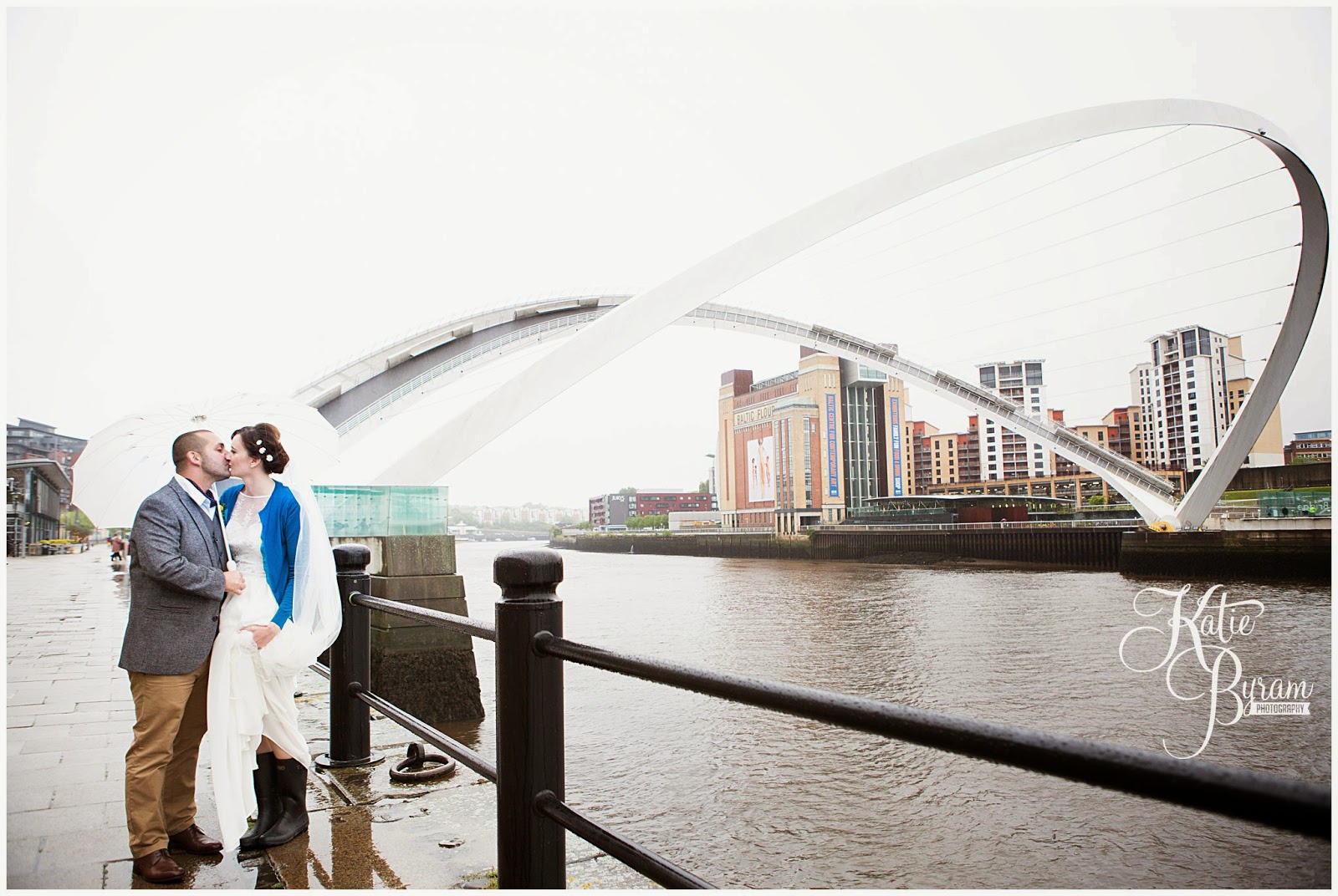In this evocative pre-engagement photograph, a couple is seen sharing a kiss under a white umbrella on the left side of the frame, set against a gray, overcast day. The couple stands on a gray boardwalk alongside a muddy, brown river, leaning gently against a metal railing that has distinct architectural features. The woman, wearing a white wedding dress partially covered by a dark blue jacket and long brown boots, has her hair done up with a delicate crown-like accessory. She holds up her dress to keep it off the wet pavement. The man, in a gray suit jacket and tan dress pants, shares the umbrella with his bride-to-be. 

In the background, a large double arch bridge with a wiring structure forms an almost heart-like shape over the river, enhancing the romantic ambiance. The photo also includes distant city buildings and a notable architectural structure labeled as the Baltic flower mill across the canal. The branding "Katie Byram Photography" is visible to the right, suggestively marking the photographer behind this intimate moment. The overall composition and subdued tones evoke a serene, love-filled atmosphere in the bustling cityscape.